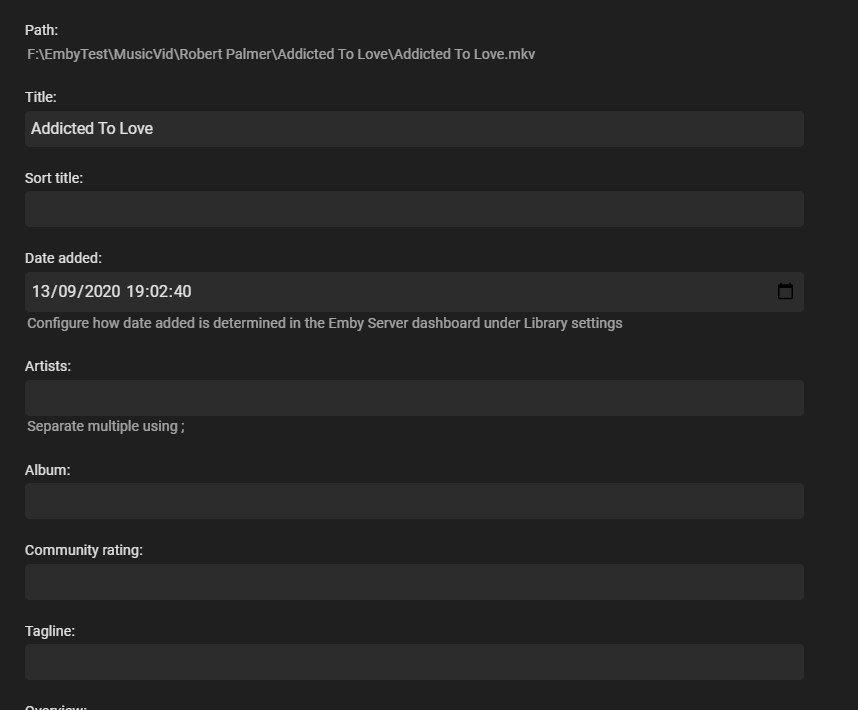### Detailed Caption

The image is a screenshot of a media management interface featuring a predominantly black background with dark gray selection bars. At the top, there is a field labeled "PATH" displaying the directory location of a file: `F:\nbtest\musicvid\robertparmer\black\addictedtolove\addictedtolove.mkv`. Beneath this, there's a "title" field containing the text "addictedtolove." Further down is a "sort title" field, which is currently empty. The "date added" field is highlighted in gray and shows the value "13/09/2020 at 19:02:40," along with a note that instructs to configure how the date added is determined in the MB server dashboard under library settings.

Continuing down, there is a blank field for "artists" with guidance to separate multiple names using a semicolon. Following this are empty fields intended for the "album name," "community rating," and "tagline," all waiting to be populated with relevant information.